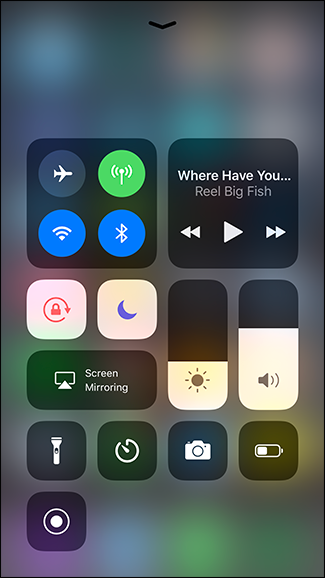The image depicts the Control Center of a recent version of iOS on an Apple iPhone, showcasing various quick-access functions. The Control Center appears as a semi-transparent overlay, with the home screen and app icons blurred in the background. It features a grid of squares and rectangles, each representing different toggles and settings. 

In the upper section, familiar options like Airplane Mode, Wi-Fi, Bluetooth, and Cellular Data are available for toggling on and off. An active media playback box occupies a portion of the screen, currently playing "Where Have You Been?" by Reel Big Fish, though the song title is cut off after "Where Have You."

Additional functional buttons are present, including Orientation Lock, Night Mode (which may relate to privacy settings), Screen Mirroring, Volume, and Brightness sliders. Other utilities visible are the Flashlight, Timer, Camera, and a partially visible battery icon indicating a charge level of approximately 35-40%.

The bottom part of the Control Center includes two rows; the first row has four buttons, while the second row has a single button resembling a bullseye – a circle with another concentric circle around it, serving an unspecified function.